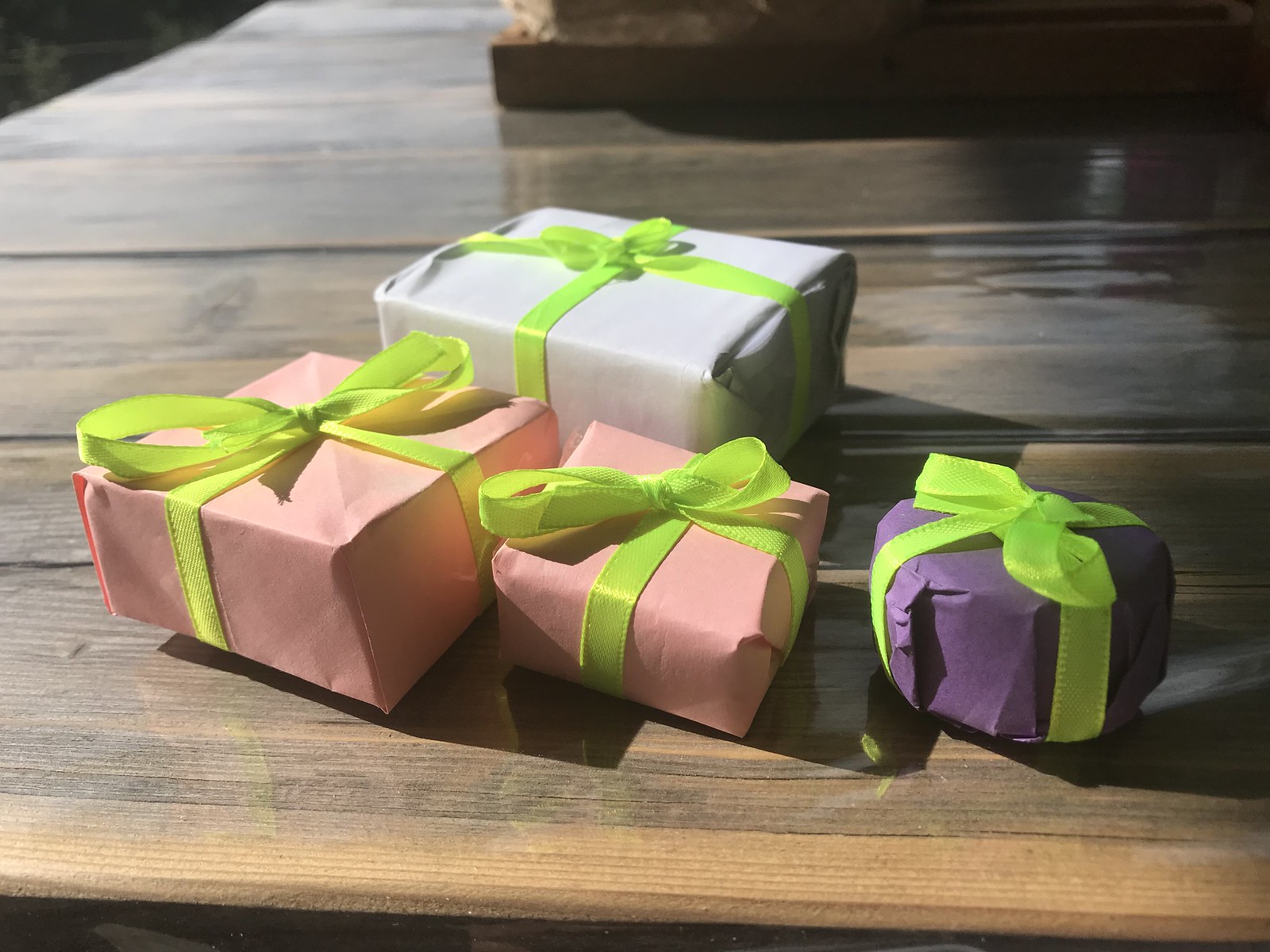In this color photograph, a medium brown wooden table with a burnished grain and individual horizontal planks serves as the setting for four gift-wrapped presents. The scene suggests a porch or deck area, enhanced by the presence of a stone wall in the top right corner and a hint of water. The table, situated in natural but dim lighting, draws focus to the central foreground where the gifts are neatly arranged. The gifts include a large rectangular present at the back, wrapped in white paper with a lime green bow, and in front of it, three smaller presents. The first, a large square package, is adorned in pink paper with a matching lime green bow. Next to it, another smaller square gift is similarly wrapped in pink paper with a lime green bow. Finally, a circular present is distinguishable by its purple wrapping paper and the same lime green bow. The repeated lime green bows contrast vividly against the varying shades of wrapping paper, making these gifts the most prominent elements in the photograph.